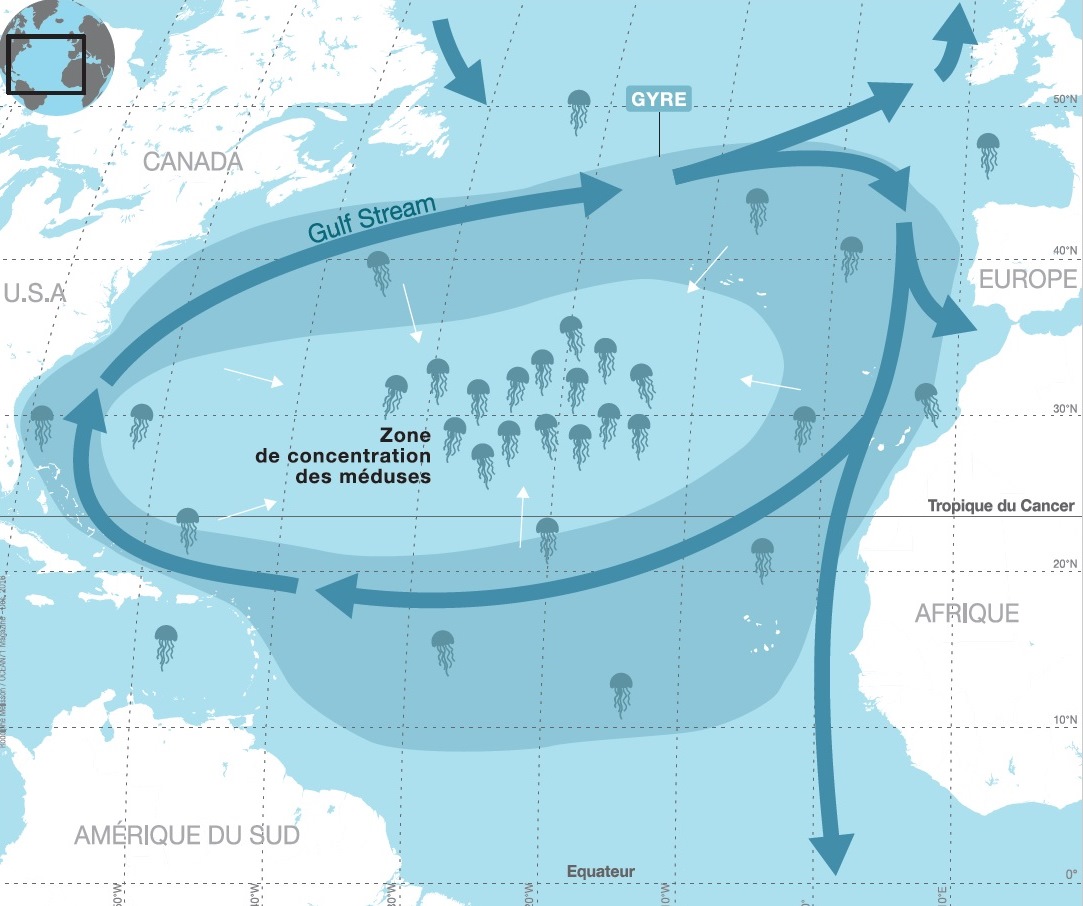The image is a detailed, color illustration in landscape orientation, depicting a map of the Atlantic Ocean. The central focus is on the Gulf Stream, highlighted with dark blue arrows forming a circular pattern around the main area of interest. This central zone, marked as "Zone de Concentración de Medusas" in black text, shows a high concentration of jellyfish, illustrated by numerous grey silhouettes scattered throughout the blue ocean. Surrounding the Atlantic, the map labels the continents and notable geographical markers: Canada and the USA to the west, South America labeled as "Amérique du Sud" to the south, Europe and Africa to the east, and the Equator ("Équateur") crossing the middle. The Tropic of Cancer ("Tropic du Cancer") is also noted. In the top left corner, a smaller globe image highlights the examined section with a black rectangle. The illustration combines elements of map cartography and infographic design to convey the migration and concentration of jellyfish within the Gulf Stream's current.